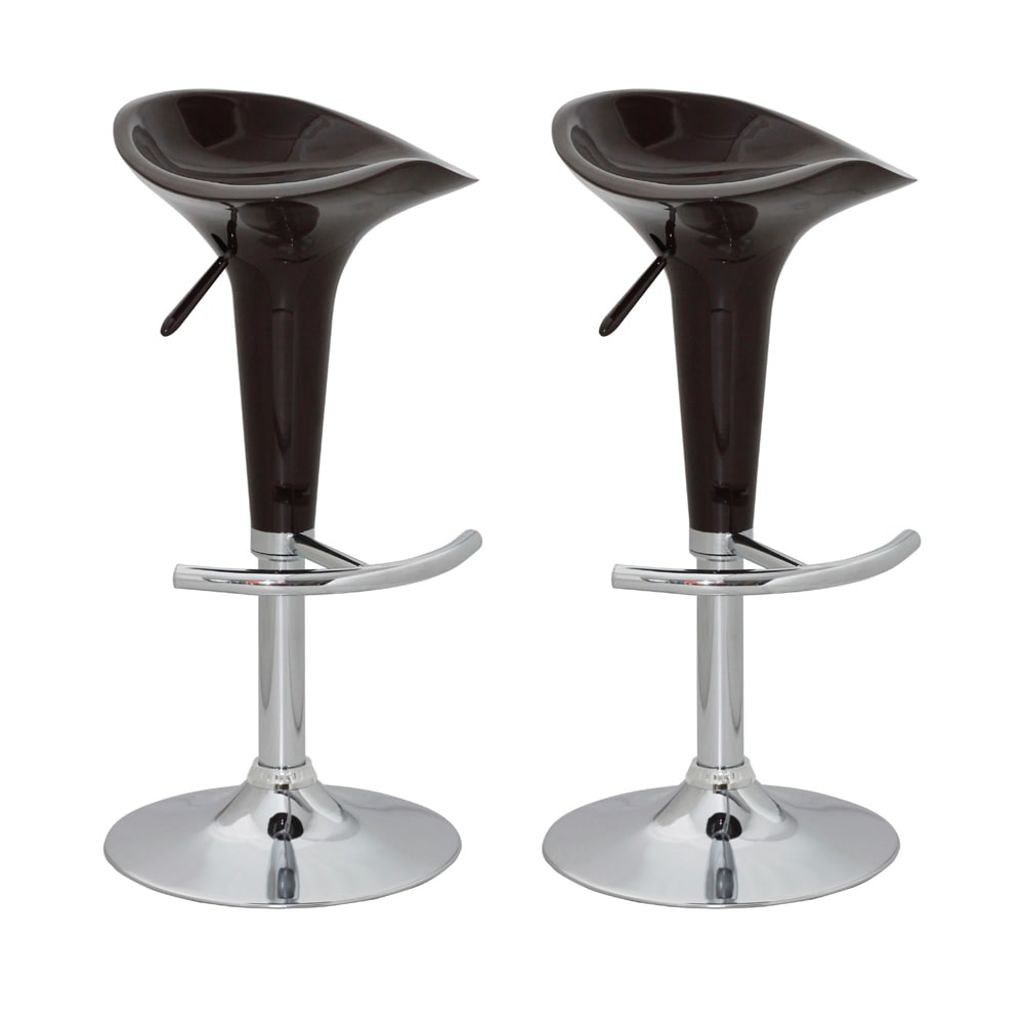This photograph features two identical bar stools, prominently displayed against a stark white background. Each stool consists of a wide, circular stainless steel base that supports a sleek, cylindrical post. Near the midpoint of the post, there is a stainless steel T-shaped footrest for added comfort. The seat itself, finished in glossy black, is ergonomically molded like a scoop or bucket to comfortably accommodate a person's hips and bottom. Additionally, a lever at the rear of each stool allows for adjustable height. Both stools are positioned side by side, their modern design accentuated by the gleaming chrome and contrasting black elements.